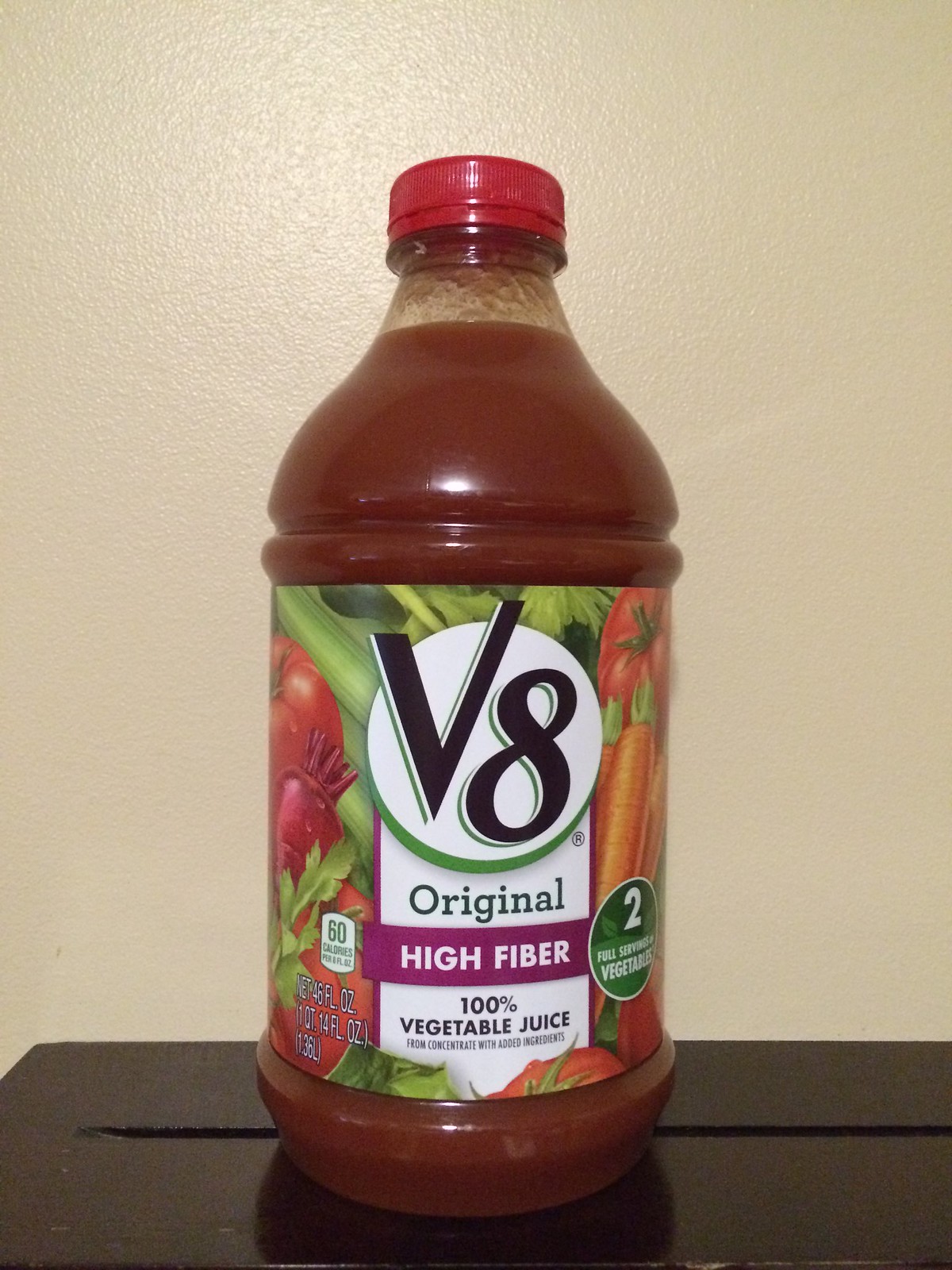The image showcases a large, brand-new, full bottle of V8 vegetable juice, prominently placed on what appears to be a dark brown wooden bench against a cream-colored plaster wall. The bottle, made of clear plastic with a narrow neck and a sealed red cap, allows a view of the rich red vegetable juice inside. Dominating the bottle is a large label adorned with vivid images of fresh vegetables, including celery, tomatoes, carrots, and beets. The label prominently features the V8 logo in large black letters, followed by the word "original" in green. Below that, a purple banner heralds "high fiber," and further down, it specifies "100% vegetable juice from concentrate with added ingredients" in black text. The label also highlights nutritional information: a green and white box on the left indicating 60 calories, and a circular green emblem on the right noting "two full servings of vegetables." Additional details about the bottle's weight are noted below the calorie information.